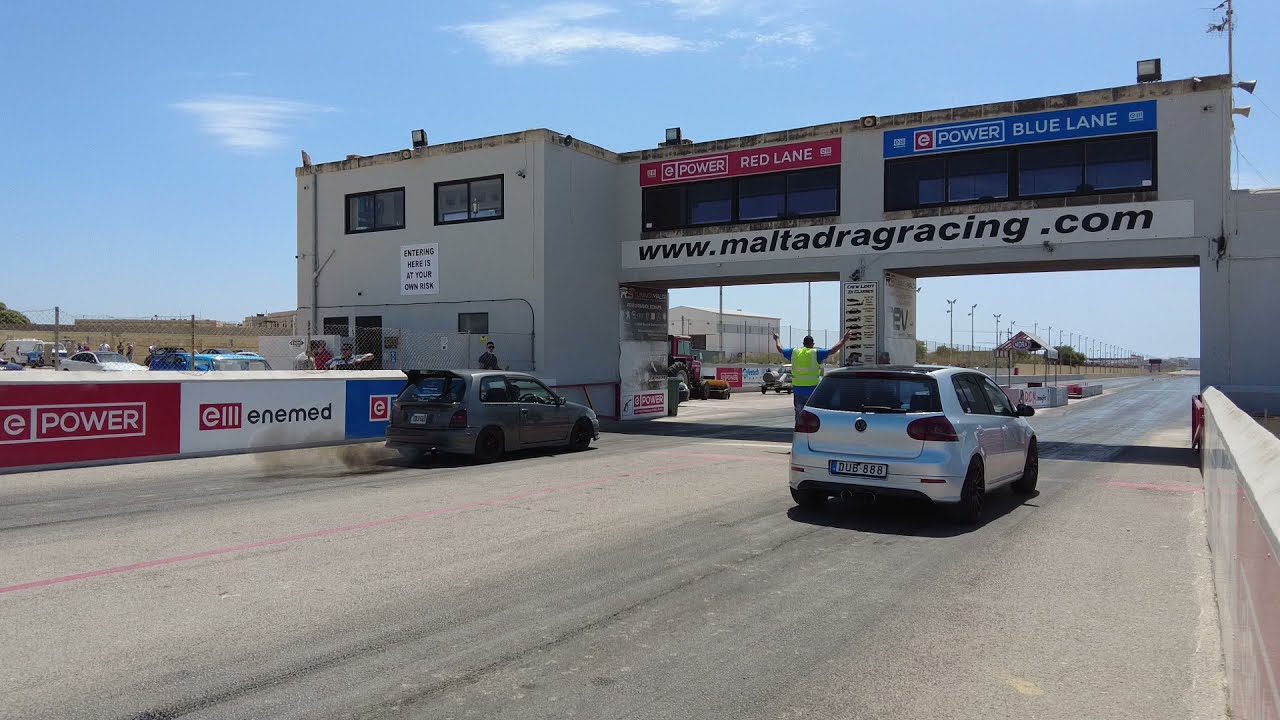The image depicts a pair of silver sedans positioned at the starting point of a raceway, set in a desert-like climate. Both cars, notable for their black wheels, are situated under an archway that spans the road, connecting two sections of the track. The car on the left emits black smoke from its exhaust, while the car on the right remains stationary. Directly in front of the vehicles stands a man in a bright green vest, arms outstretched. He is situated under a building that arches over the racetrack, bearing the website www.maltadragracing.com. The building features windows on the upper level and displays a red banner labeled "Power Red Lane" on the left and a blue banner labeled "Power Blue Lane" on the right. To the left of the track, there is a two-story, light cream-colored building with two upper-floor windows, along with visible cars and people in the distance. Adjacent to the man and the track is a barrier marked with the text "EII ENEMED" and the word "Power." Shadows cast by the overhanging building fall across the ground, and a row of lights separates the two tracks. Overhead, the sky is mostly blue, dotted with light white clouds.